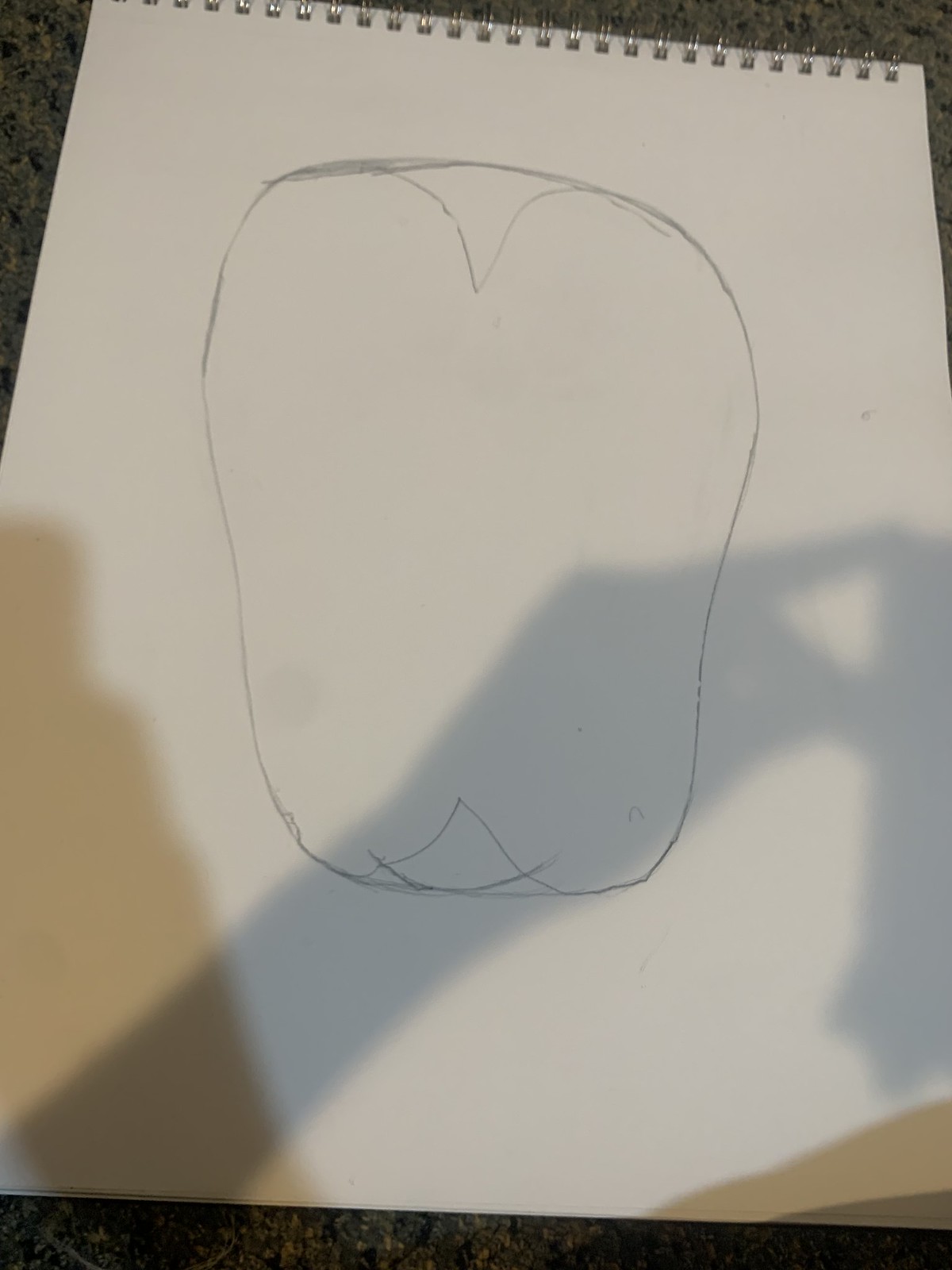The image depicts a simple pencil sketch on a white sketch pad, which is bound by a spiral at the top, indicating it's part of a flip-over notepad. The paper is slightly tilted to the left, resting on a black countertop. The drawing itself is a somewhat rounded oval shape with indentations at the top and bottom. The top indentation begins to form the shape of a heart, while the bottom features an indentation resembling that of a tooth or a chin. The sketch appears to be an attempt at drawing a heart within a circle, with the heart's top and bottom sections partially outlined. Additionally, the photo captures distinct shadows, showing the outline of the photographer’s hand and possibly their nose, as they lean forward to take the picture with a smartphone.